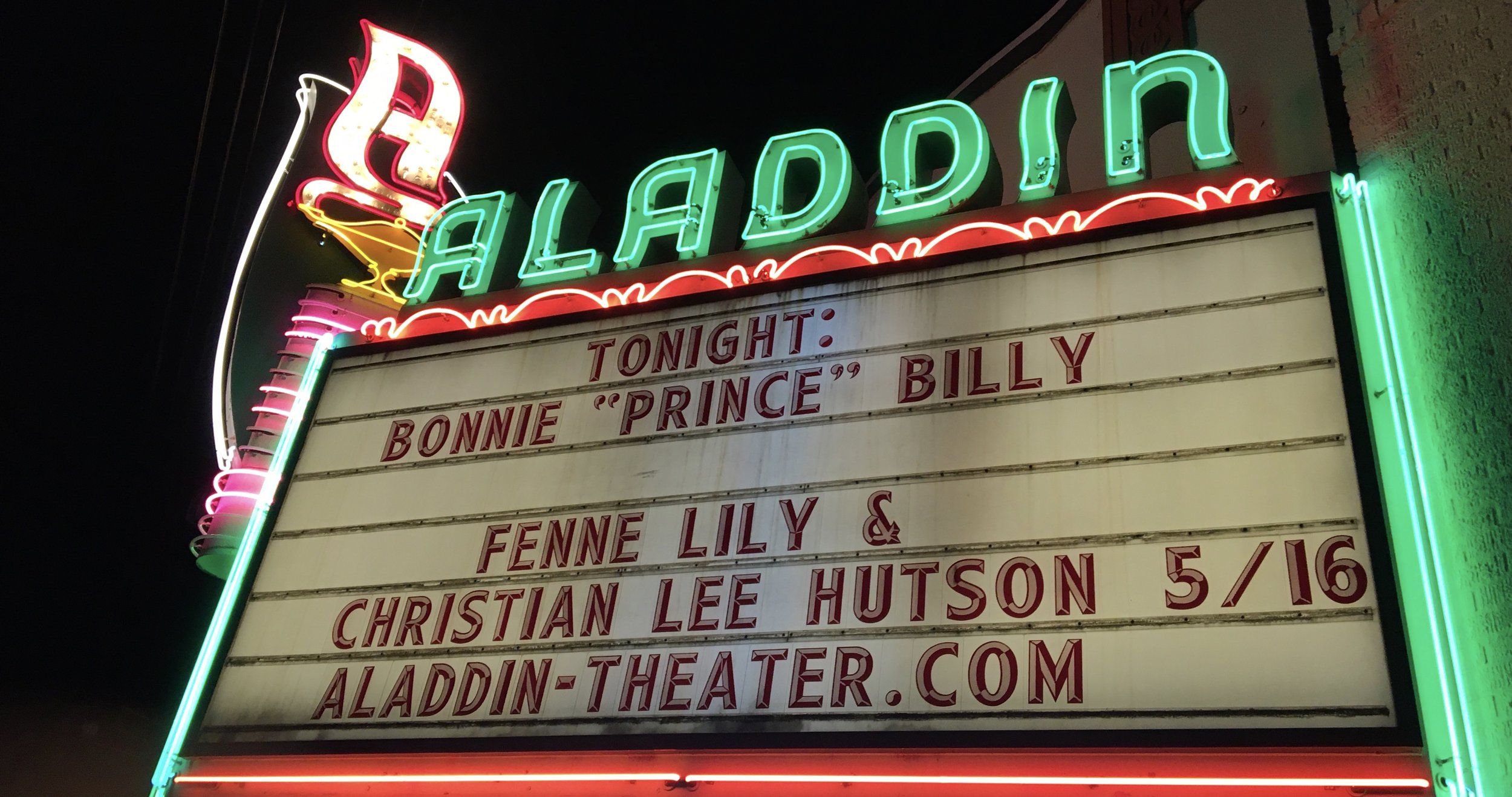The image captures a vibrant billboard of the Aladdin Theater, illuminated with various neon lights. The top of the billboard prominently displays the word "ALADDIN" in teal-colored neon lights, shining brightly in all capital letters. Beneath "ALADDIN," the marquee reads: "Tonight, Bonnie 'Prince' Billy," followed by "Finn Lillie and Christian Lee Hudson, 5/16," indicating a performance date of May 16th. The bottom of the marquee lists the website "Aladdin-theater.com."

The billboard also features additional neon lighting accents. On the right, there is a teal neon light, complemented by a reddish-orange neon light below. Although harder to see from the angle, the left side also contains a teal neon light. At the top left corner of the billboard, a vivid letter "A" emerges from a golden genie lamp, accented in an orangish-reddish hue, adding a touch of magical whimsy to the theater’s display.